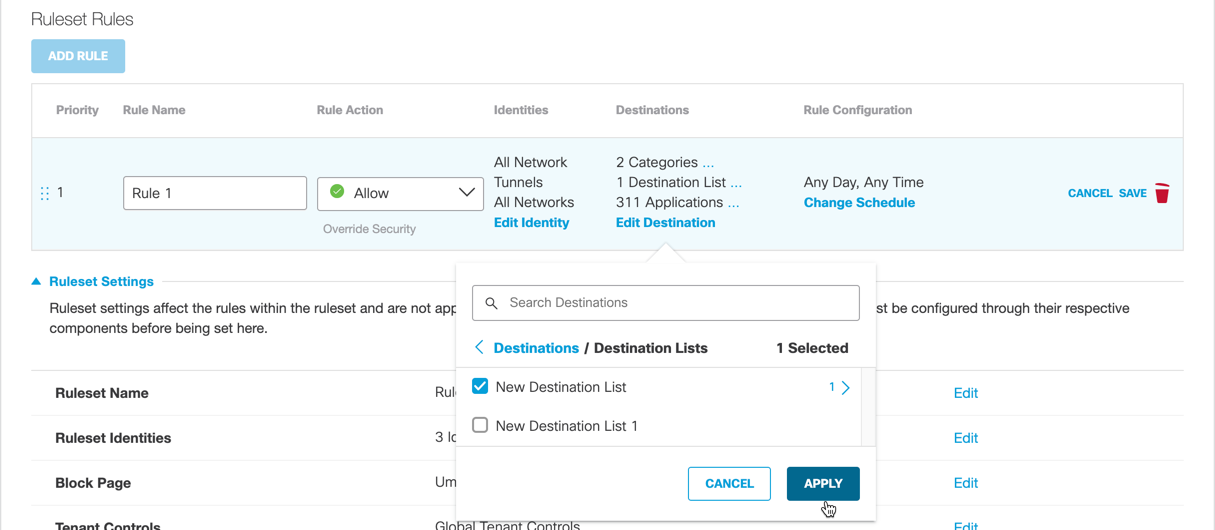On this webpage, the background is predominantly white. In the top left corner, there's bold black text, albeit somewhat difficult to read, likely stating "RULIST RULES" followed by "RULIEST RULES". Below this, a light blue box with white text displays the option "ADD RULE". Under it is a long rectangular section labeled with columns titled "PRIORITY", "RULE NAME", "RULE ACTION", "IDENTITIES", "DESTINATIONS", and "RULE CONFIGURATION". Here, users can type in and configure various rule options, with buttons for "Cancel" or "Save". Beneath these settings is another interactive section featuring a drop-down box labeled "DESTINATION", "DESTINATION LIST", alongside options to "Cancel" or "Apply" the selected destination. Additional fields are labeled "RULIST NAME", "RULIST IDENTITIES", "BLOCK PAGE", and "TENANT CONTROLS". Overall, this website appears to be a tool for creating and managing different rules, likely meant for application in various scenarios or systems.